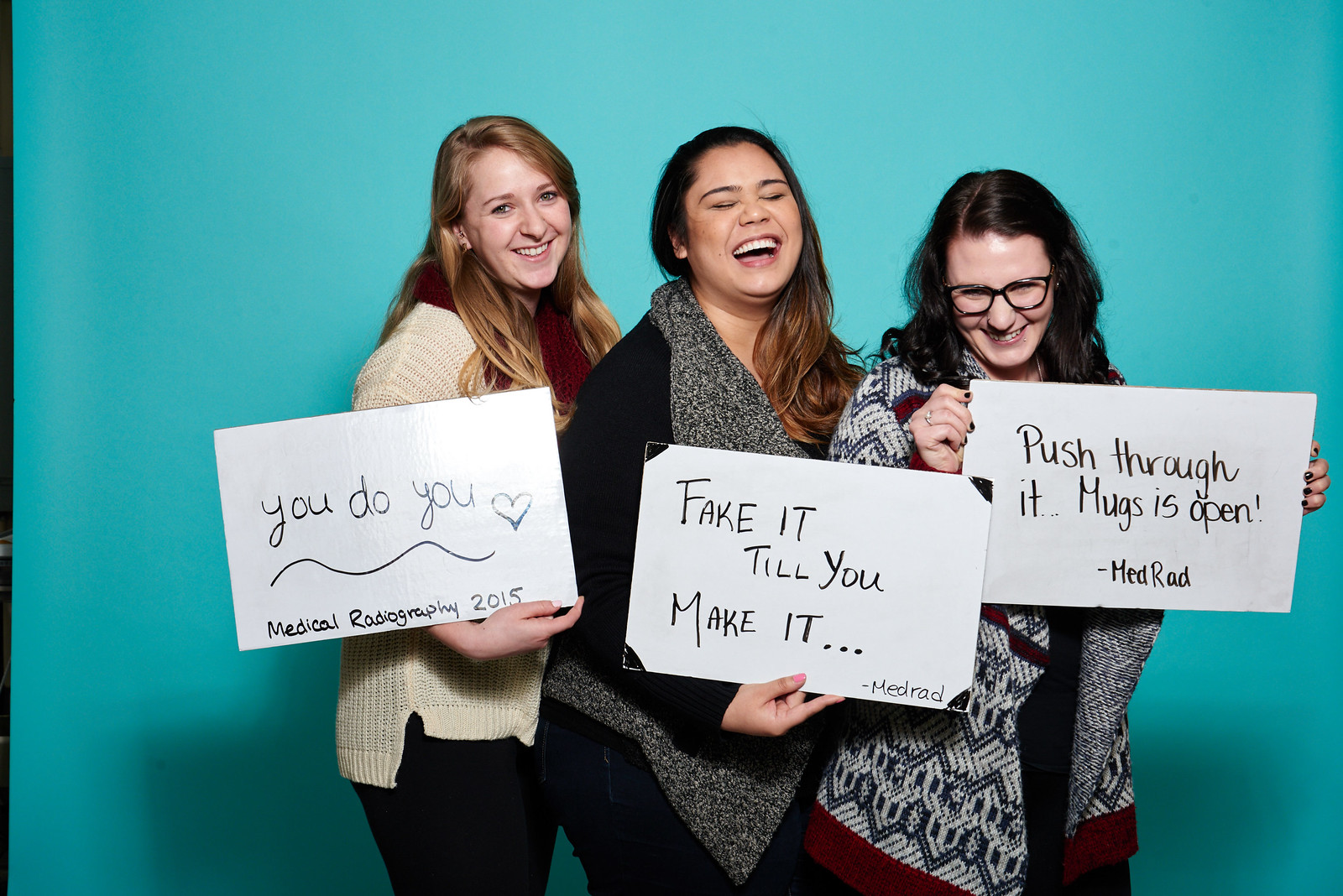The image features three women standing side by side, smiling and laughing against a light blue background. Their shadows are softly cast on the wall behind them, and each holds a small whiteboard with handwritten messages. On the left, a blonde woman in a cream-colored sweater holds a sign that reads, "You do you," with a small heart underneath, followed by "Medical Radiography 2015." The woman in the middle, with dark hair and wearing a black sweater, holds a sign that says, "Fake It Till You Make It," signed "MedRAD" in the lower right corner. The woman on the right, who has long dark hair, glasses, and is wearing a red and black knit sweater, holds a sign that reads, "Push Through It," followed by "Mugs Is Open!" and signed "MedRAD" at the bottom. Their joyful expressions and casual posture suggest a moment of camaraderie and encouragement, possibly celebrating a milestone or achievement in their medical radiography studies.